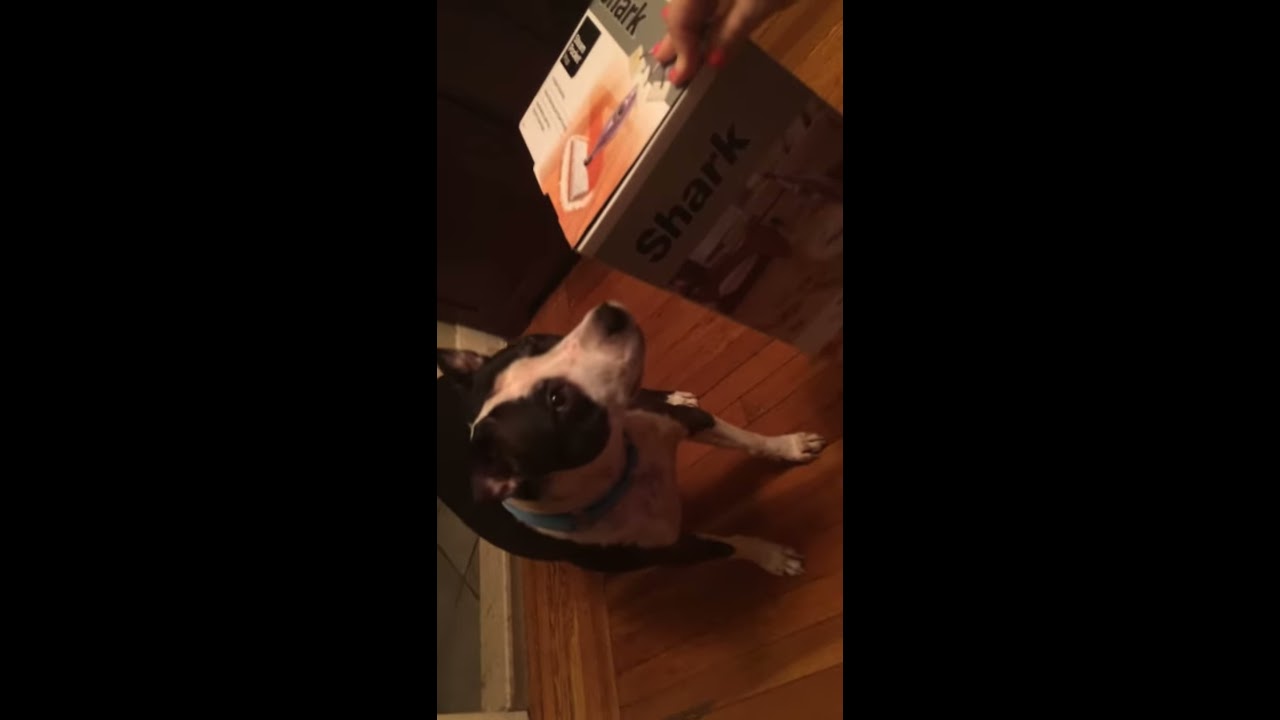The image is an indoor, vertically-oriented photograph, centered against a black landscape background. It features a small to medium-sized dog, approximately 45 pounds, with a white coat accented by either black or very dark brown spots. Uniquely, the photo is positioned sideways, making the dog's feet point to the right and its head to the left. The dog stands on a hardwood floor next to a gray box with a white top, which prominently displays a picture of a flat-headed mop, suggesting it is a container for a floor-cleaning device like a Swiffer. A small portion of a person's hand touches the corner of the box. Behind the dog, a white baseboard is visible, and the overall lighting in the image leaves parts of the box in shadow, contributing to a realistic, representational aesthetic typical of pet portraiture.